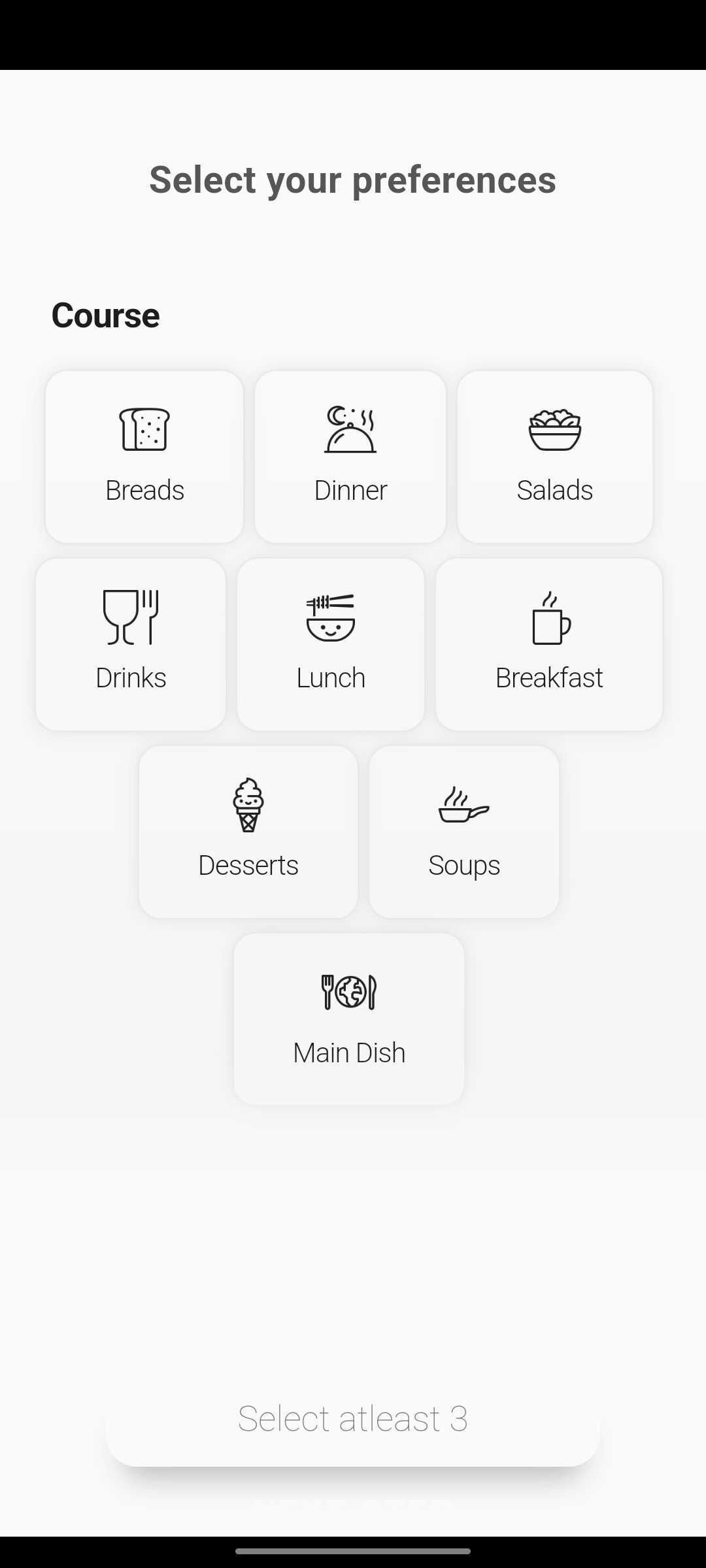The image is a rectangular screenshot, seemingly captured from a mobile phone interface. Along the top of the image is a thick, solid black bar without any text. The bottom section features a thinner dark black bar with a smaller, shorter, gray bar centered within it. 

Between these two bars, the main section of the screenshot has a light gray background adorned with dark gray text and icons. At the very top of this section, a heading reads "Select your preferences" in sentence case. Slightly below this heading, aligned to the left, another title reads "Course."

The content below this title is organized into a series of button icons arranged in rows. The first row showcases three icons: a loaf of bread representing "Breads," a covered dish with rising steam symbolizing "Dinner," and a bowl of salad for "Salads." The second row also contains three icons: a beverage glass for "Drinks," a sandwich for "Lunch," and a sunny-side-up egg for "Breakfast." The third row features two centered icons: a slice of cake for "Desserts" and a steaming bowl for "Soups." Finally, positioned solo and centered at the bottom of the button set, is an icon displaying a plate with a fork and knife, labeled "Main Dish."

Beneath these buttons is some empty space followed by a grayed-out button at the very bottom, which reads "Select at least three."